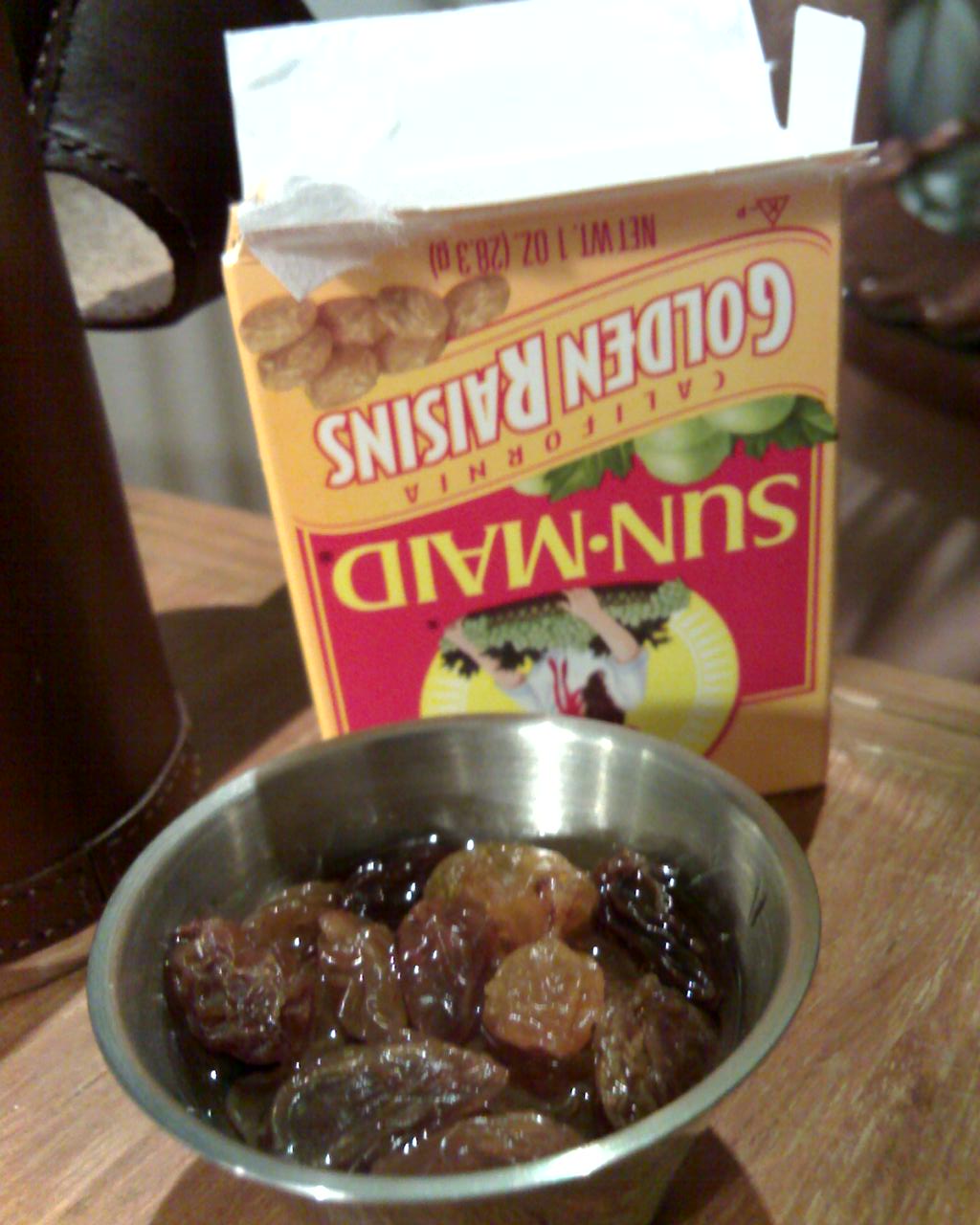This is a vertically aligned rectangular image taken on a medium brown wooden table or countertop. At the bottom of the picture sits a small, shiny metallic bowl filled with golden raisins, which range in color from light beige to dark brown and appear slightly wet. The shape of the bowl is reminiscent of a small dipping sauce container, tapering off towards the bottom. Behind this bowl, towards the top of the image, is an upside-down box of Sun-Maid Golden Raisins. The box, primarily yellow, features a red rectangle with the "Sun-Maid" logo in yellow letters at the center. In the logo, a woman is depicted holding a bushel of grapes. The box was opened from the bottom and remains open. To the left of the bowl and box, on the table surface, is a blurry, cylindrical brown object. In the background, a brown or gray tiled surface is visible but out of focus.